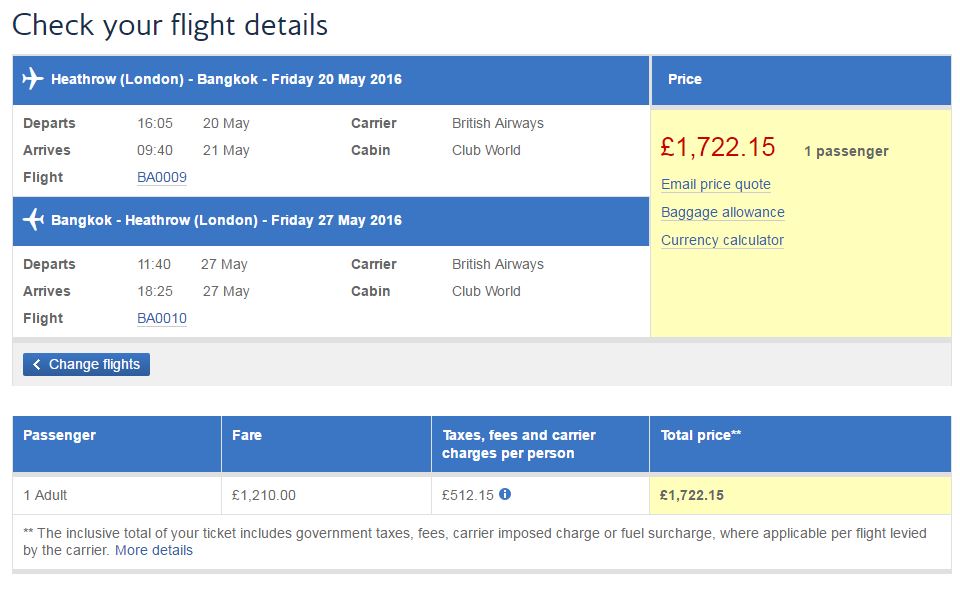**Detailed Caption:**
The image depicts a detailed screenshot of flight booking information for a round trip between Heathrow, London, and Bangkok. 

In the top left-hand corner, a header reads, "Check Your Flight Details," followed by a blue bar containing the first leg of the journey: 
- **Route:** Heathrow, London to Bangkok
- **Date:** Friday, 20 May 2016
- **Departure Time:** 16:05 (20 May)
- **Arrival Time:** 09:40 (21 May)
- **Flight Number:** BA 0009
- **Carrier:** British Airways
- **Cabin:** Club World

Below this, another blue bar indicates the return leg of the journey: 
- **Route:** Bangkok to Heathrow, London
- **Date:** Friday, 27 May 2016
- **Departure Time:** 11:40 (27 May)
- **Arrival Time:** 18:25 (27 May)
- **Flight Number:** BA 0010
- **Carrier:** British Airways
- **Cabin:** Club World

On the right-hand side of the image, a price bar is displayed at the top, followed by a beige box. The box contains the total one-passenger price: 
- **Price:** £1,722.15

Below the price, there are several options for:
- **Email Price Quote**
- **Baggage Allowance**
- **Currency Calculator**

Further down, there is a blue button labeled "Change Flights," and beneath it, additional fare details are provided in a blue bar:
- **Passenger Fare:** £1,210
- **Taxes, Fees, and Carrier Charges per Person:** £512.15
- **Total Price:** £1,722.15

The layout provides a comprehensive overview of the booking details, including flight times, costs, and additional services.